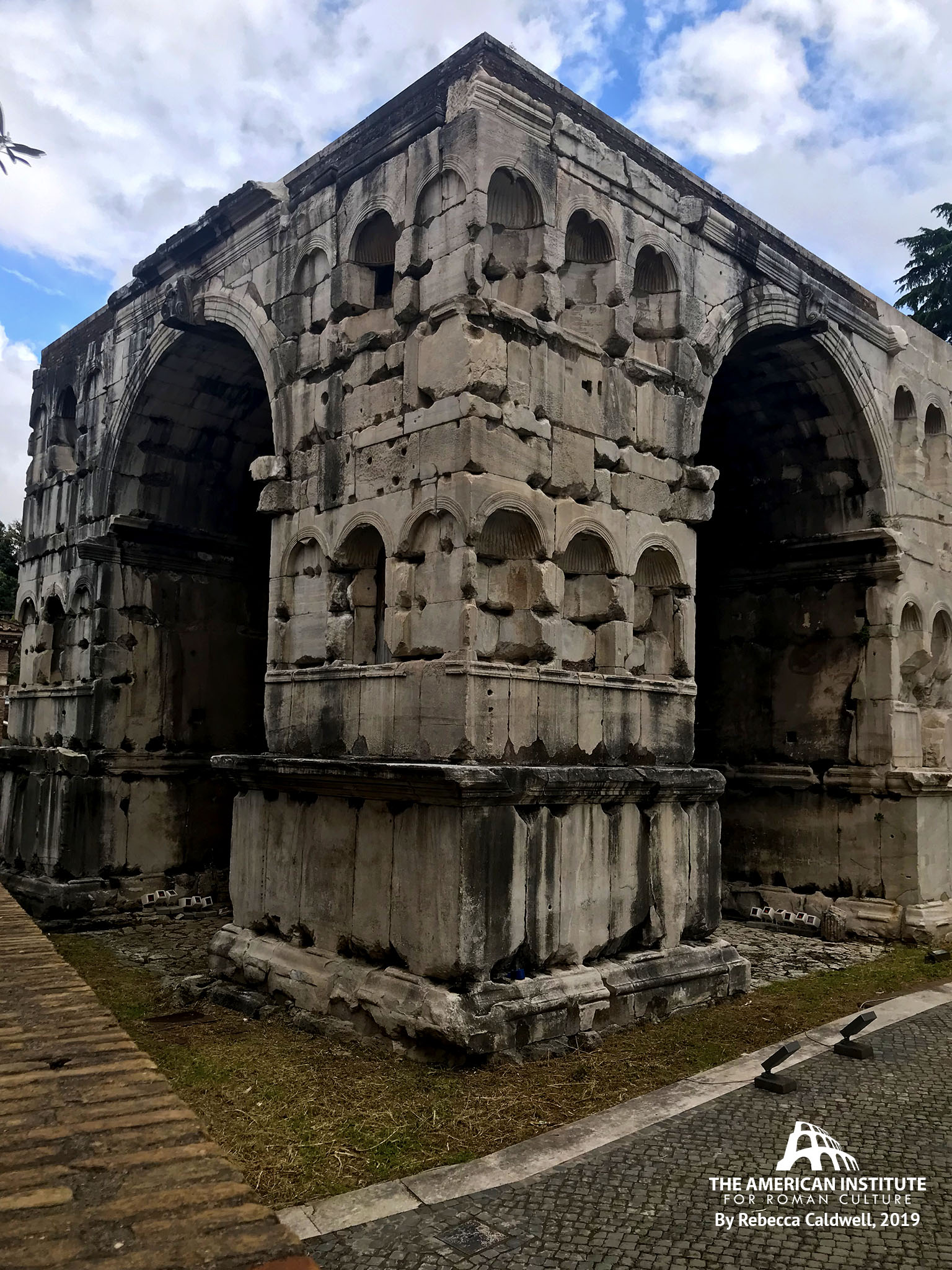The image, attributed to the American Institute for Roman Culture by Rebecca Caldwell in 2019, showcases a historic Roman building that exudes the charm of ancient architecture. This tall, weathered structure is made from what appears to be cement or stone and features two large, rounded archways extending almost to the top of the edifice, suggesting it has withstood the test of time. The building sits on a patch of grass that looks dead and short, interspersed with areas of mulch or dirt. In front of the building, there is a brick road and a stone walkway, both adding to the aged ambiance of the scene. To the right, a cobblestone pathway leads towards the structure, flanked by two light fixtures that look like solar lights. The overall appearance of the building is worn, with blackened areas along its brown surface indicating weathering, giving it a venerable yet enduring presence. Above, the sky is a clear blue with scattered white clouds, enhancing the timeless beauty of this ancient Roman architectural marvel.